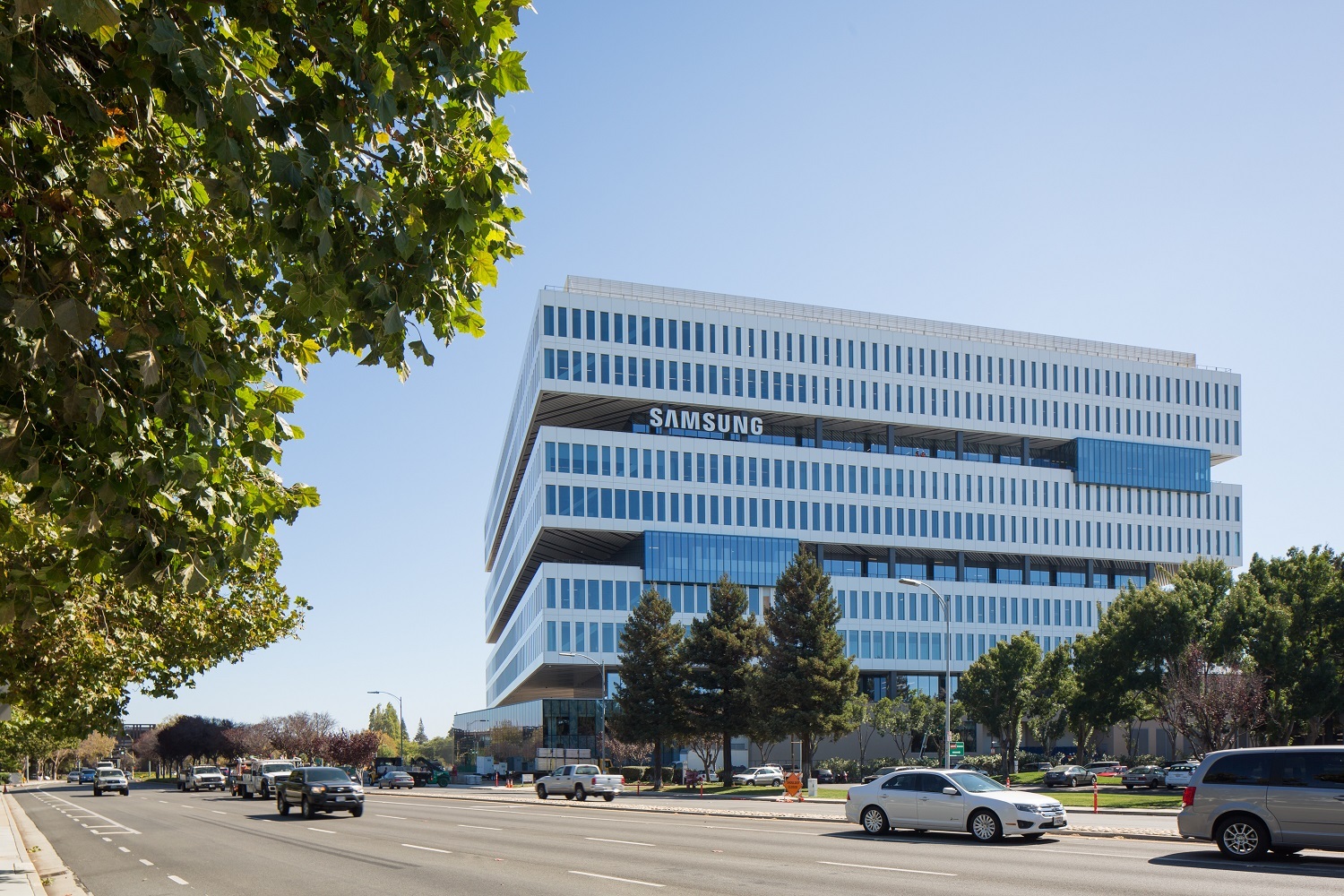In this vibrant urban scene, the focal point is a striking, multi-storied Samsung commercial building. The architecture features a "layer cake" design, with alternating white and dark glass slats giving it a modern, blocky appearance. Dominating the skyline, the building is at least 12 stories tall, with the prominent Samsung logo displayed on the middle-left section of the structure. 

The scene is captured on a bright and sunny day, highlighting the building's crisp lines against a completely clear blue sky. Below the imposing structure, a bustling four-lane highway, divided by a concrete median, is visible with numerous cars and trucks moving in both directions. Bike lanes are also present, catering to the urban commute.

On the left side of the photograph, a mature tree with lush green foliage overhangs the road, adding a touch of nature to the urban landscape. Additionally, a series of trees line the sidewalk in front of the Samsung building, providing a green buffer between the building's lawn and the busy roadway. The overall clarity of the image invites viewers to immerse themselves in the dynamism of city life juxtaposed with modern architectural elegance.